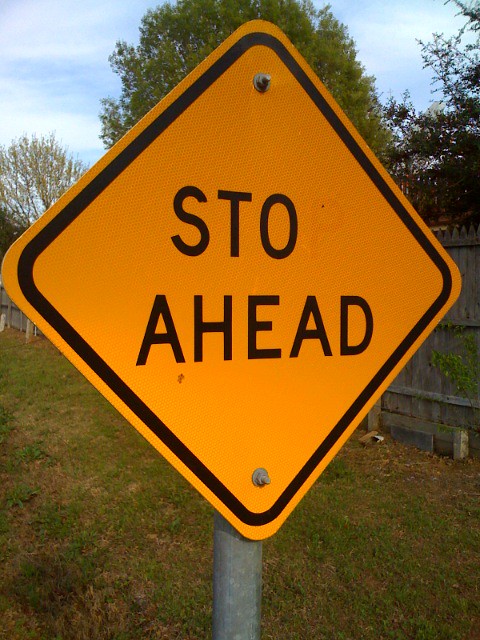This is an outdoor photograph featuring a yellow, diamond-shaped street sign with a black border. The sign is mounted on a galvanized steel pole with two bolts securing it. The text on the sign should read "STOP AHEAD," but the 'P' is faintly visible as if it has been erased, leaving "S-T-O" followed by "AHEAD" in capital letters. The sign appears weathered and is situated on a grassy strip. Behind it, there is a somewhat weathered wooden privacy fence, and further in the background, a few trees and a sky with wispy clouds are visible.